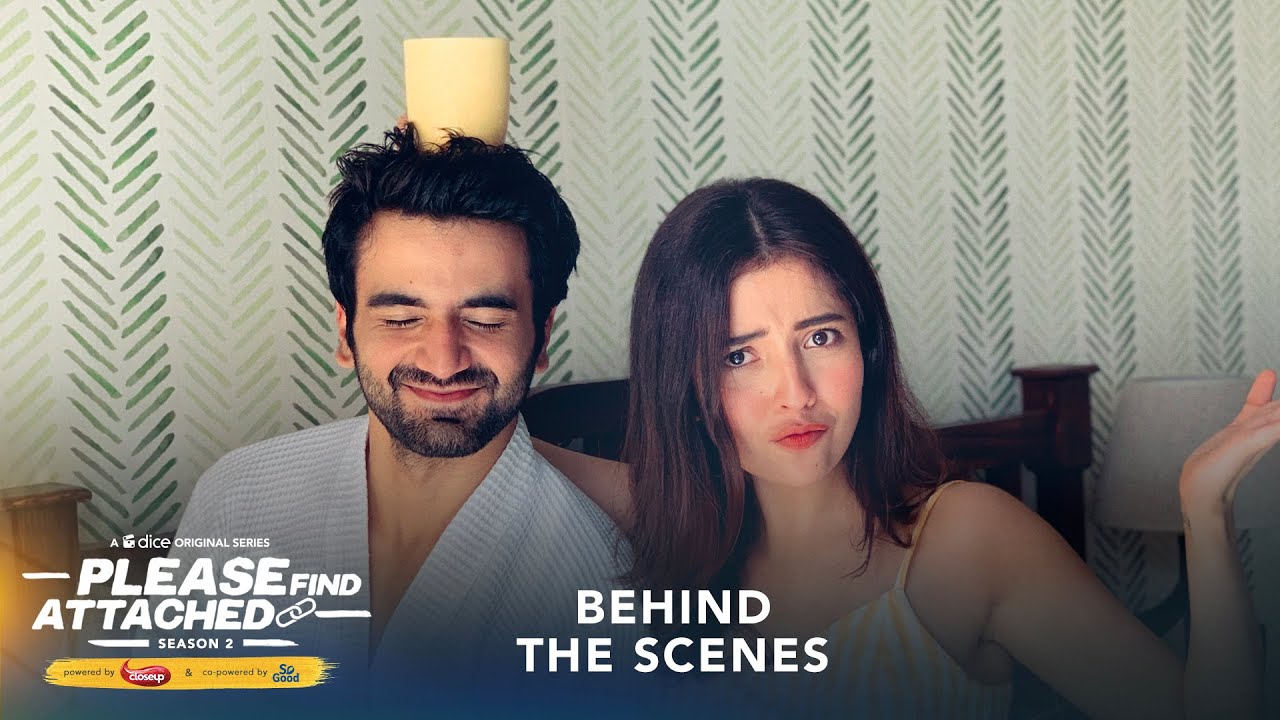This is a promotional behind-the-scenes image from the DICE original series "Please Find Attached," Season 2. The image features a couple, a man and a woman, sitting closely together, both with dark hair and lighter skin. The man, sporting a closely-trimmed beard and wearing a robe, has his eyes closed, smiling with a content expression. The woman, wearing thin-strapped pajamas and pale pink lipstick, has a goofy, confused look while staring directly at the camera. Intriguingly, she also has a cup perched on top of his head and her arm affectionately draped around him. The textured wallpaper in the background showcases interesting fins and angles or a pattern of green and brown leaves extending upward. The image text includes "A Dice Original Series, Please Find Attached, Season 2," emphasizing its behind-the-scenes nature.